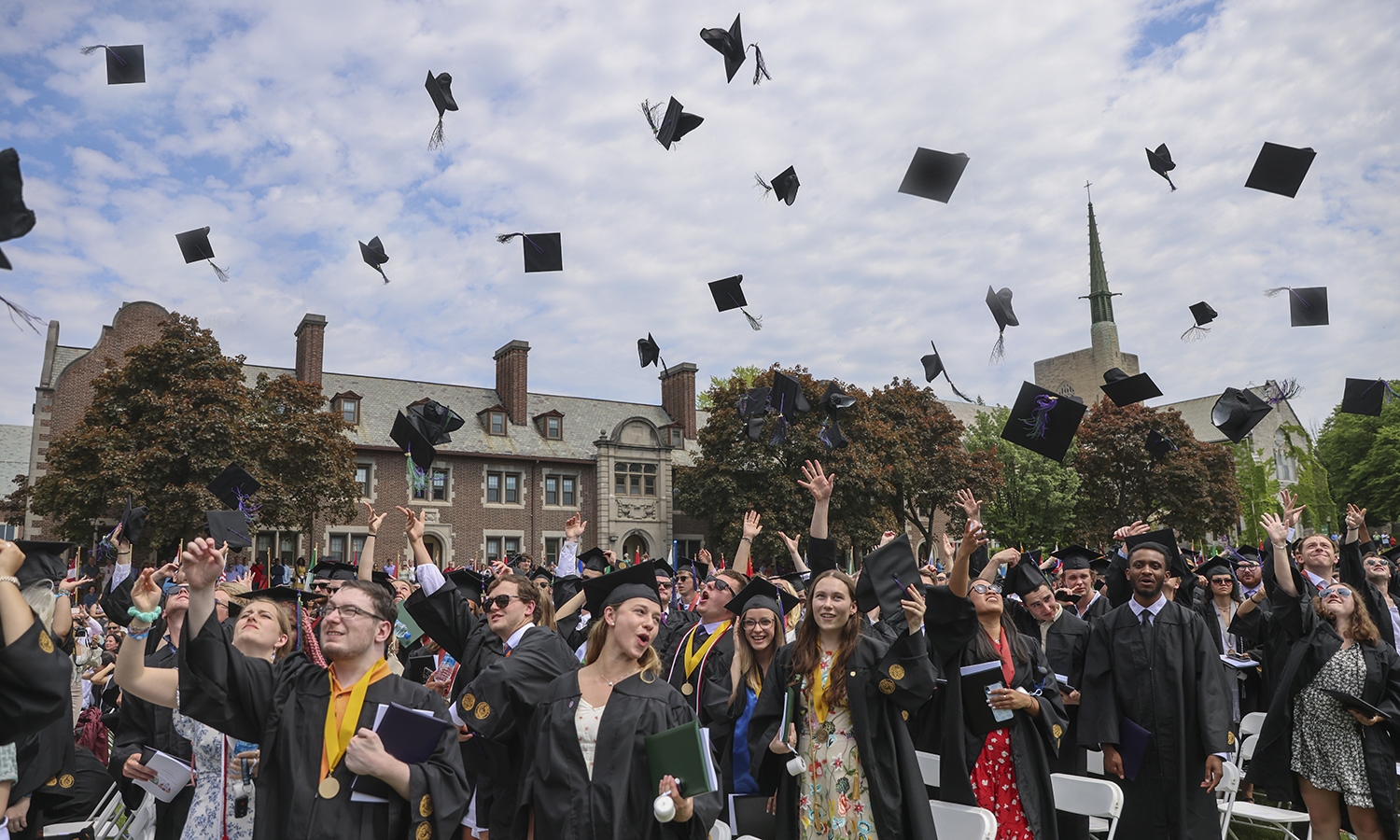The photograph captures a lively college graduation ceremony set outdoors on a mostly cloudy day. A sea of graduates, wearing iconic long black robes, stand up from their white chairs in rows and jubilantly throw their black caps with blue tassels into the air. Many of the students, some adorned with medals and honors cords, can be seen cheering and reaching their hands upwards, clearly in high spirits. The scene is framed by an academic setting: dark brown brick buildings typical of a college campus, with one large rectangular building featuring three chimneys and a gray roof. To the right, a building with a tall, pointed structure capped by a cross stands prominently, adding a touch of architectural grace. Short trees with dense foliage dot the landscape between the buildings and the graduates. The upper portion of the image showcases a beautiful sky with patches of clouds, adding depth and a sense of open celebration to the moment.